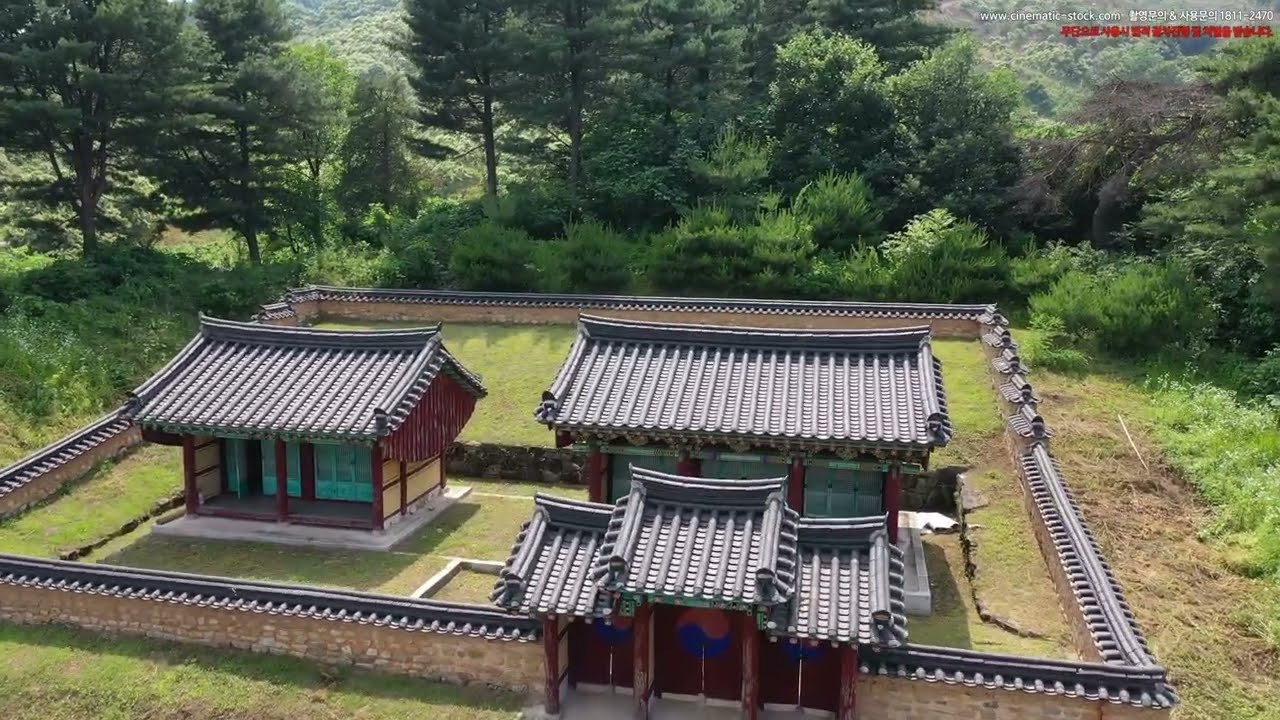The photograph captures a serene, daytime outdoor scene featuring a traditional Asian temple complex. At the heart of the image are two small, one-story temples centered within a beige stone-walled courtyard. The temples boast dark metal shingled roofs and red painted wooden grids with light yellow panels on their sides. The gated entrance to the courtyard, positioned at the right-hand corner, has a distinctive three-door design that matches the shingled roofs. Surrounding the courtyard are lush, tall green trees that add a vibrant contrast to the scene. The background reveals a mix of natural brush and mountainous terrain, enhancing the remote, tranquil atmosphere. On the image, "www.cinematic-stock.com" is printed in white, followed by Korean characters and the numbers "1811-2470." Below this, additional Korean text appears in red. The overall palette features greens, browns, blues, yellows, reds, blacks, and grays, contributing to the detailed and culturally rich depiction.